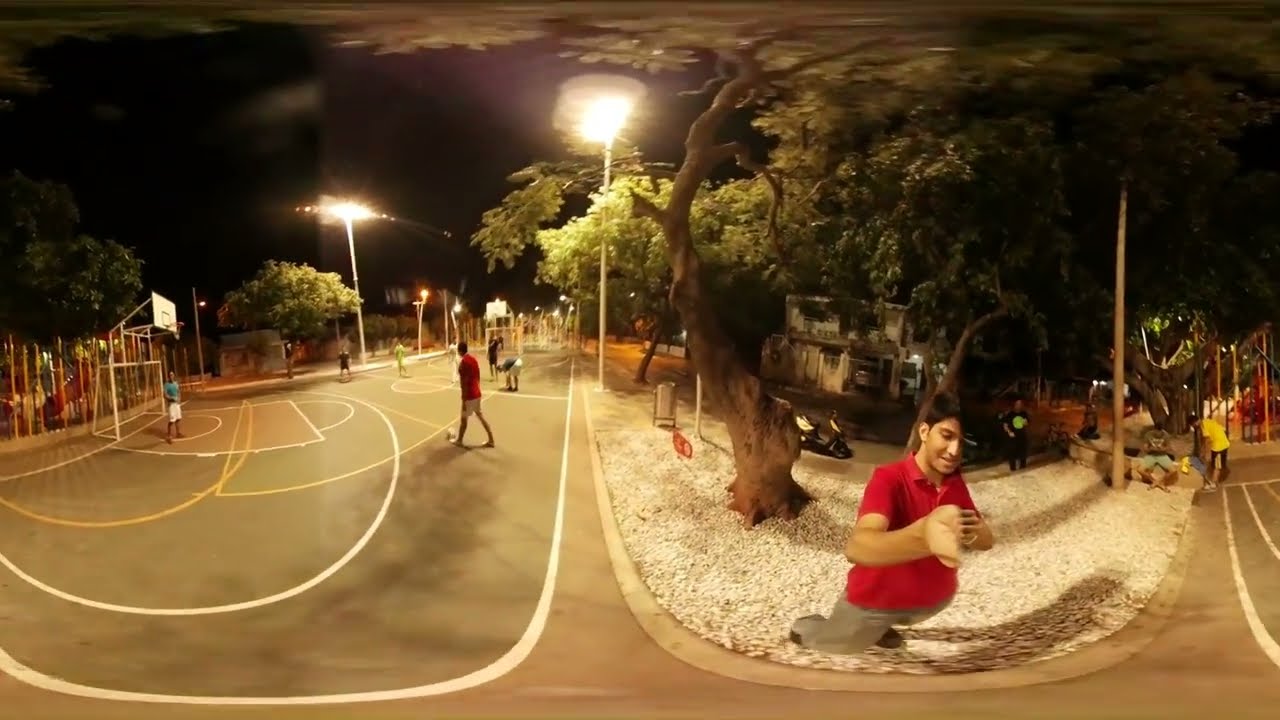In this distorted fisheye lens photo, taken at night, a man with dark hair wearing a red polo shirt, gray pants, and running shoes stands near the bottom center-right of the image, looking down and holding a yellow object in his hands. He is positioned on a gravel path, surrounded by a multifaceted outdoor scene. To his left is a vibrant play area featuring a basketball court with a soccer net behind the hoop, where individuals are engaged in what appears to be a hybrid game or multiple activities simultaneously, including soccer and basketball. Illuminated by three bright streetlights on poles, the scene is bustling with various people scattered across the area. One notable moment captured is a person wearing red and white shorts actively kicking a soccer ball. The background includes distorted views of trees and buildings, adding to the surreal ambiance. To the right center, a motorbike and several bicycles are visible, complementing the lively and dynamic environment of this park-like setting.